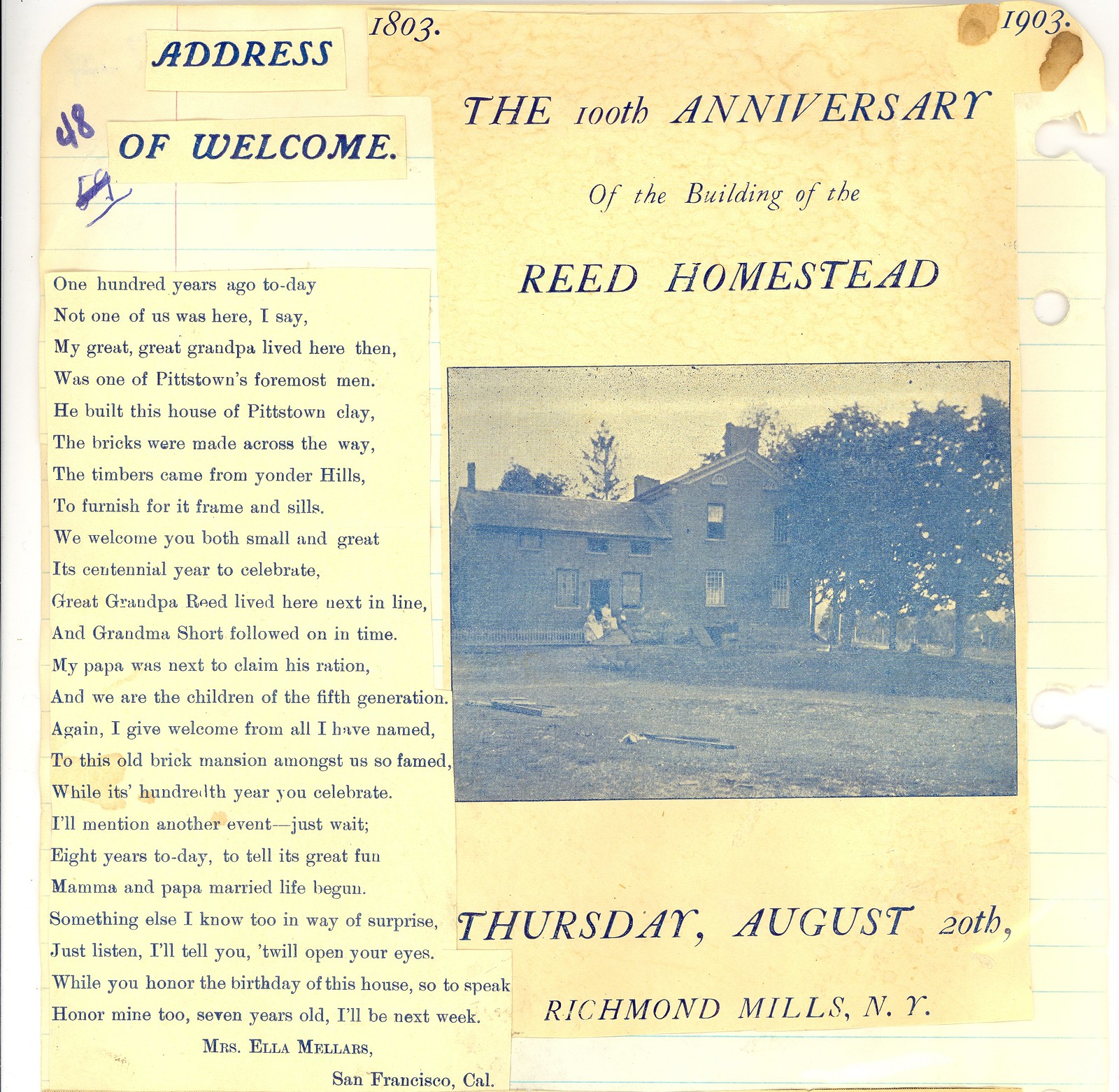This image captures a yellowed page from a notebook, which appears to be aged and water-stained. The notebook page features an article titled "Address of Welcome" marking the 100th Anniversary of the Building of the Reed Homestead, dated Thursday, August 20th, in Richmond Mills, New York. The page includes a column of text on the left, detailing a familial and historical recount of the Reed Homestead's significance, beginning with "100 years ago today, not one of us was here, I say." The narrative celebrates the lineage of the Reed family, mentioning various ancestors and their contributions to the homestead, and culminating in a personal anecdote from Mrs. Ella Miller of San Francisco, California. On the right side of the page, there is a black-and-white photograph of a large, two-story farmhouse surrounded by trees, possibly with a couple of people sitting on the porch and a grassy pathway leading up to the house. At the bottom of the photo, the date and location are clearly inscribed: "Thursday, August 20th, Richmond Mills, New York." The page also bears handwritten scrawls, including the years "1803" and "1903," and some numbers that have been struck through.